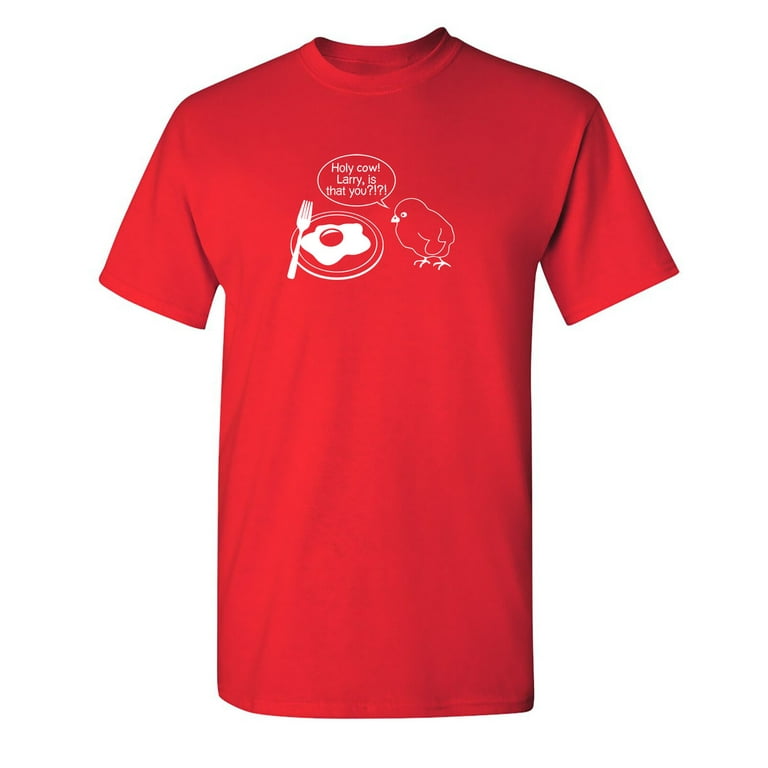This is a product image of a deep bright red, short-sleeved t-shirt with a crew neck displayed against a plain white background, as if set up for an online clothing store. Central to the shirt’s design is a humorous and detailed illustration: on the right side of the shirt is the white outline of a small, chubby bird characterized by clear lines depicting its feet, beak, and eye. The bird, situated to the right, appears to be speaking through a white text bubble that reads, “Holy cow, Larry, is that you?!”

To the left of the bird, there is a depiction of a clear plate bearing an egg cooked sunny side up, with its yolk colored the same deep red as the shirt, and a fork is placed beside the plate. The quirky and cute arrangement suggests that the bird is astonished and looking at the egg, possibly hinting at a humorous dialogue. The t-shirt’s playful design makes it a standout piece, perfect for a lighthearted addition to anyone's wardrobe.